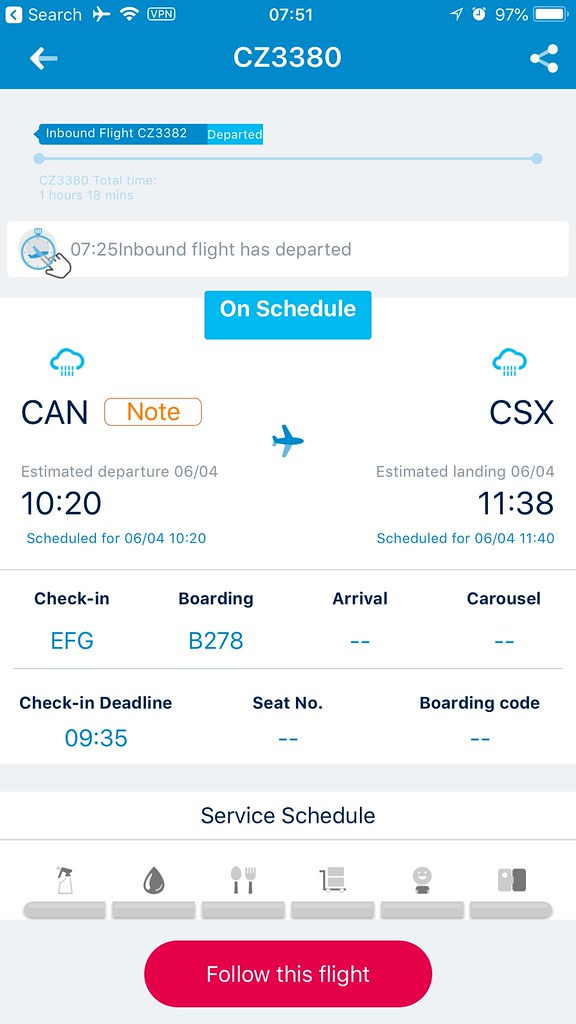A detailed screenshot from a mobile device displays an open flight application against a blue background. At the top, a header with white text provides a search bar, alongside icons for a plane, Wi-Fi, and VPN. The status bar shows the time, an alarm icon, and a battery indicator at 97%. The main content at the top displays the flight number "CZ3380," under which the status reads "725 inbound flight has departed on schedule." The departure location "CAN" (presumably Guangzhou Baiyun International Airport) has an estimated departure time of 2023-10-20 06:04. In the middle of the screen, a graphic of an airplane outlines the flight path.

To the right of the plane graphic, the arrival location "CSX" (Changsha Huanghua International Airport) is noted with an estimated landing time of 2023-10-20 11:38. Below these details, check-in instructions indicate an "EFG" section for check-in, a boarding gate "B278," but the arrival terminal and baggage carousel information are yet to be determined as they show a dash. The check-in deadline is listed as 09:35, with the seat number and boarding code also noted with dashes, signifying that they are yet to be assigned. At the bottom, navigation options include "Service Schedule" and "Follow This Flight."